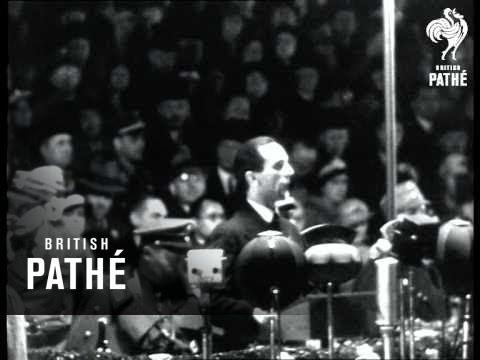This is a black-and-white image, resembling an old photograph or historical TV broadcast, marked by a distinctive style indicative of the early 1900s. The scene captures a notable press conference or speech, with a white man with slick-backed hair standing centrally in the foreground, addressing the audience. He is speaking into several microphones of various shapes, including circular, square, and oval, which are positioned towards the bottom right corner of the image. The background reveals a densely packed crowd, seated in what appears to be a stadium or large audience hall, all facing the speaker. The image bears the text "British Pathé" in white, with a watermark in the bottom left corner and a rooster logo alongside identical text in the top right corner, emphasizing its historical and archival nature.